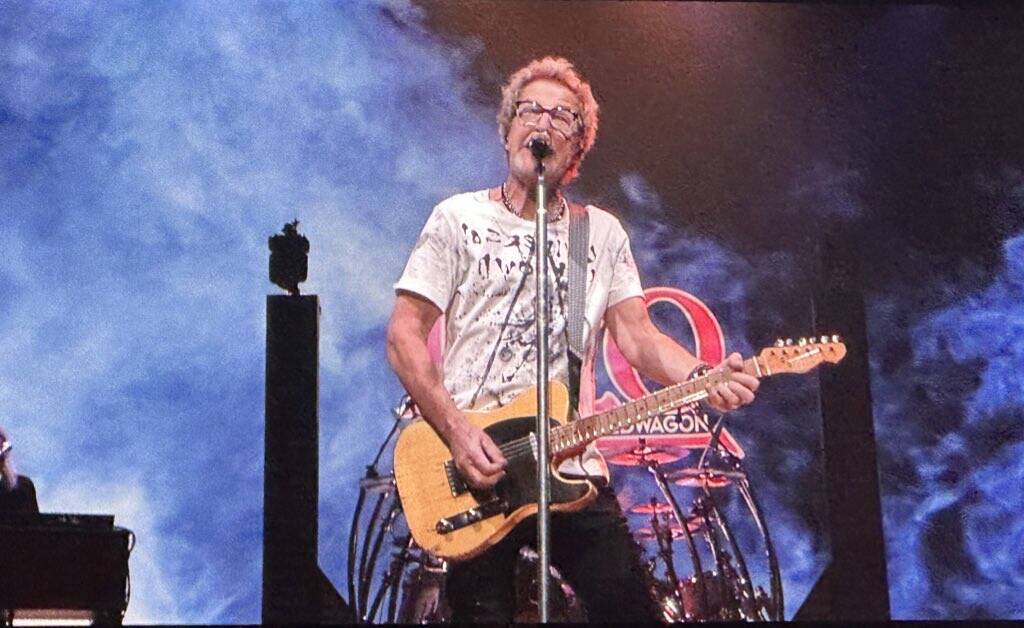The rectangular photograph, likely a still from a video, features Kevin Cronin, the singer of REO Speedwagon, performing in a concert setting. The image centers on Cronin from the knees up, who is positioned in front of a silver microphone stand equipped with a black microphone pointed towards his mouth. He is dressed in black denim jeans and a white short-sleeved shirt adorned with assorted black characters. A chain necklace hangs around his neck, and he is wearing glasses. Amidst a smoky and foggy atmosphere tinged with blue and white hues, Cronin grips an electric guitar with a natural wood faceplate. Behind him, partially obscured by the smoke, symbols and a drum set are visible, along with fragments of the band's logo projecting in red. To the left, another piece of musical equipment is faintly seen in the shadows. The backdrop and staging elements, including two black pillars, frame the performer, highlighting the dynamic ambiance of a live indoor concert.